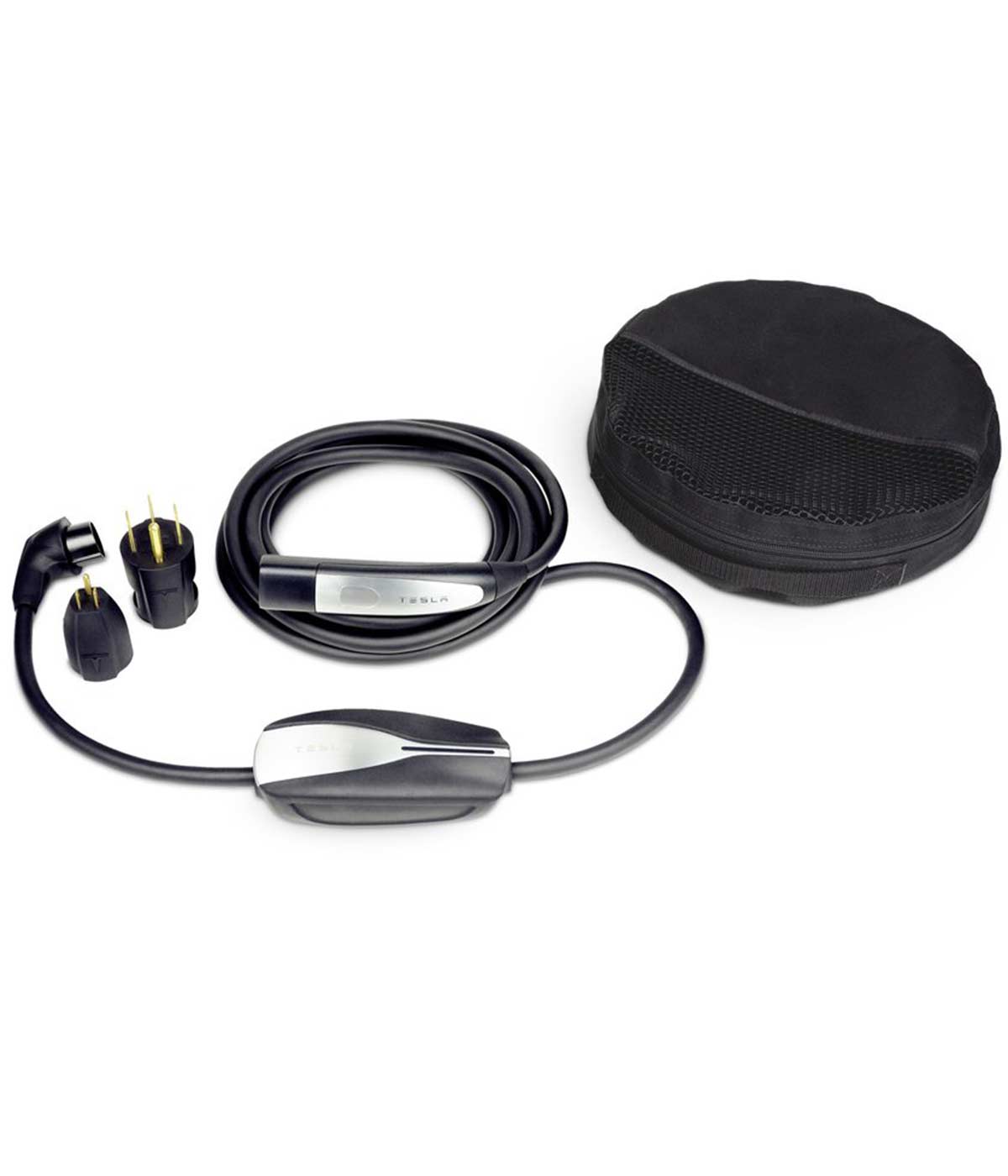The image depicts a Tesla-branded electronic charging cable designed for use with Tesla vehicles. This black cable features a silver logo on one end that reads "Tesla," suggesting its specific application for Tesla cars. The cable is equipped with two different types of connectors, likely different plug types for various outlets. Next to the cable, there is a round, black carrying case with a textured, possibly leather exterior and a black handle, designed for easy transportation and protection of the cable. The setup is displayed against a white background, highlighting the cable's length and coiled nature.